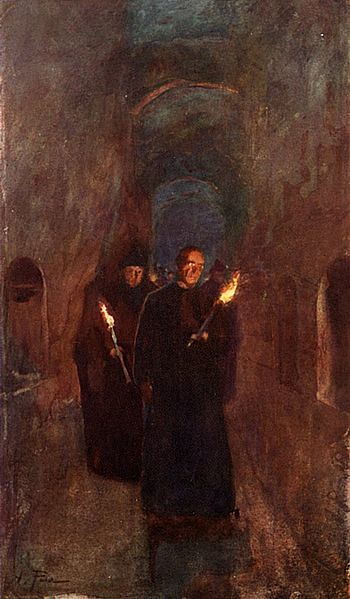The painting depicts a group of robed men, likely monks of Caucasian heritage, walking through a narrow, arched stone tunnel that resembles catacombs. The men, at least three in number, are holding flame torches that illuminate the otherwise dark setting. The figures are clad in long, dark, floor-length robes, with the leading individual being bald and possibly wearing glasses, while two men behind him don pointy black hats. The tunnel features tall, grayish-brown walls with domed alcoves on either side, suggesting it may have been carved out of stone or constructed to mimic such a setting. Arch support beams span the top of the tunnel, adding to the desolate, foreboding atmosphere. This watercolor painting seems to evoke a religious or historical context, heightened by the solemnity and uniformity of the figures and their monastic appearance.